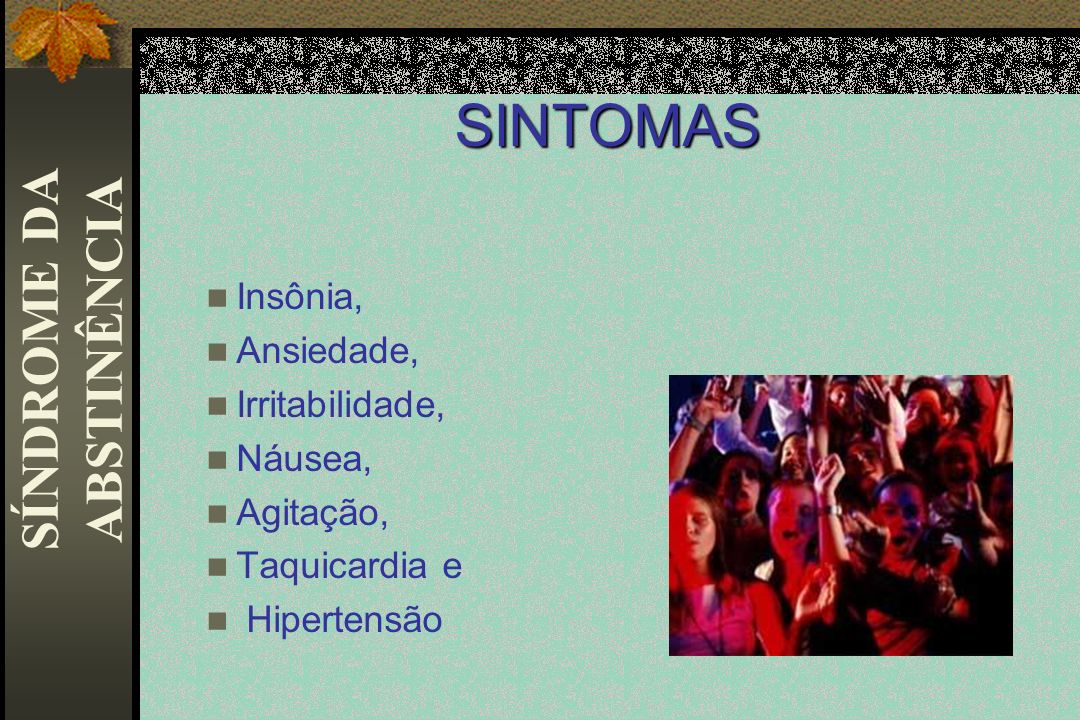The image is a colorful infographic, resembling a PowerPoint presentation slide, focused primarily on graphics and text in a different language. Dominating the top-middle section, the word "Sintomas" is prominently displayed in dark blue against a light green background. On the left side, the text reads "Sindrome da abstinencia" in white within a gray rectangle. Below this title, a list of symptoms is presented in bullet points, featuring words such as "Insania," "Incididae," "Irritability," "Nausea," "Legitical," "Tachycardia," and "Hypertensia" in various languages like Portuguese and possibly Latin or Spanish. 

In the bottom right corner, there is a small rectangular photographic image depicting a crowd of young people, likely at a concert, illuminated by red and purple lighting. The overall color scheme of the infographic includes shades of black, white, brown, orange, yellow, and red, creating a vibrant and visually engaging presentation.